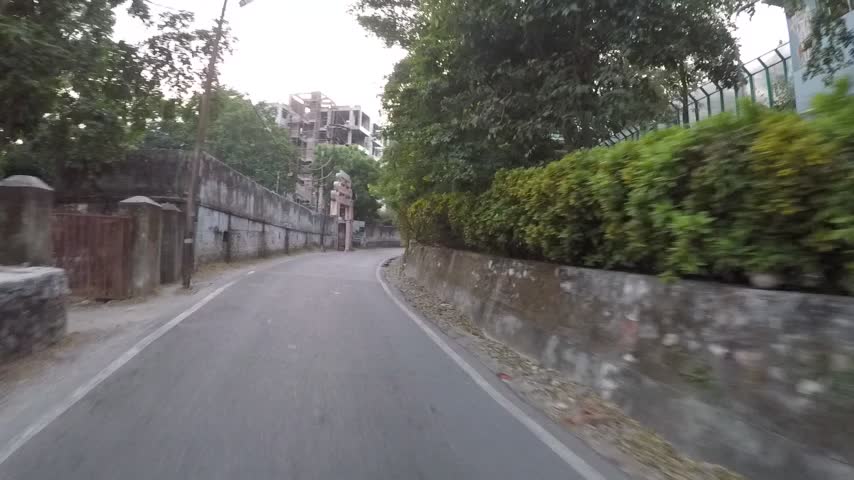This detailed picture captures a curving, one-lane road running through what appears to be a residential area of a city or town. The light gray asphalt road features white lines marking both its edges. On the right side, a four-foot-tall concrete barrier runs along the entirety of the road, topped by dense green bushes and interspersed with occasional barbed wire. Above this barrier, there's a fence, behind which stands a large tree. Near the curve of the road, on the right, glimpses of a white building are visible.

On the left side of the road, there is a walkway lined with occasional concrete structures and a series of red-brown brick walls with gray concrete caps. Trees, power lines, and a brown post with a streetlight are observed, giving a sense of the surrounding urban environment. Further left, additional foliage and a metal fence with prominent concrete pillars provide a backdrop.

In the distance, past the bend, a tall, modern apartment building, possibly under construction, rises above the surrounding trees and structures, creating a notable juxtaposition against the more traditional elements of the area. The road ultimately curves away, disappearing behind trees, which adds to the scenic and somewhat secluded ambiance of the setting.